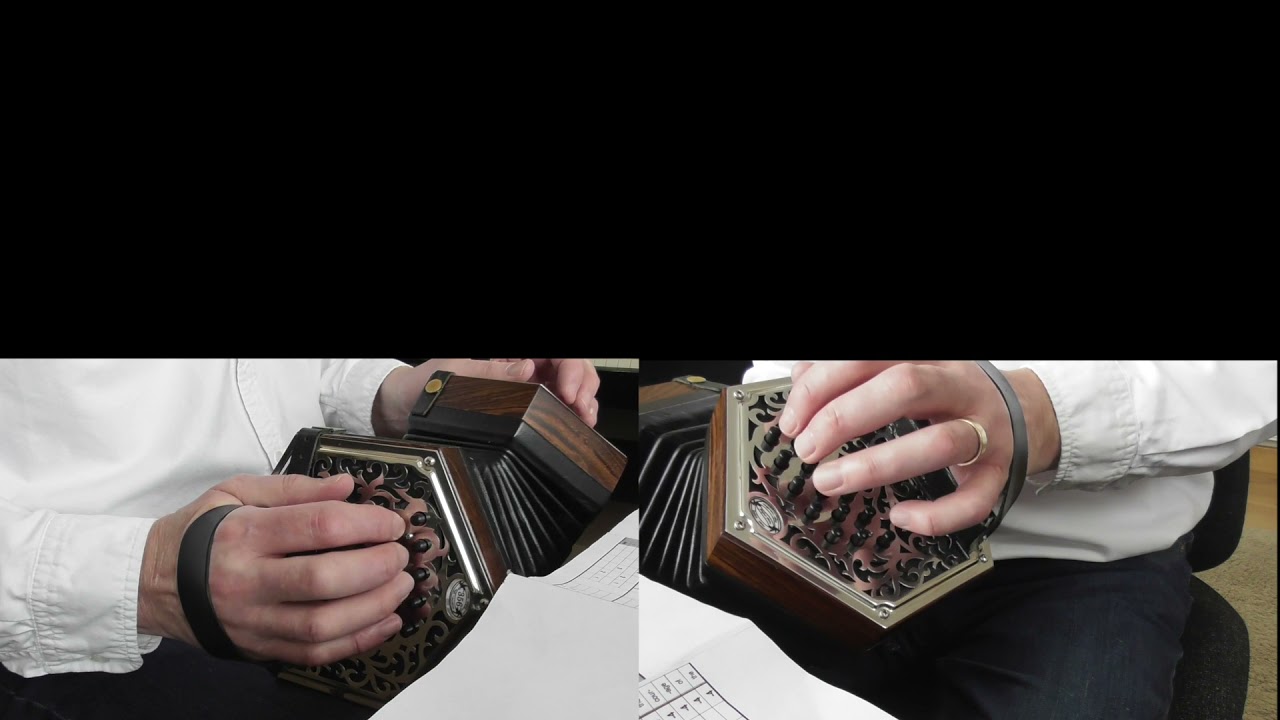The image consists of two distinct photographs placed side by side, occupying the lower half of the entire picture, while the upper half is covered by a solid black bar. Each photograph showcases a person holding a small, stylistically attractive accordion with intricate designs, possibly featuring mother of pearl inlay. Both individuals appear to be male, with visible wedding rings on their left hands, suggesting they might be married. They are dressed in white, long-sleeved button-down shirts. The person on the left is seen from the torso down to their black pants, and the one on the right is similarly shown from the torso, with an additional white paper included in each image—possibly with printed images. Both are seated, and the angle suggests the person on the left is oriented towards the left while the person on the right faces towards the right. The dual photographs emphasize the detailed craftsmanship of the accordions and the formal attire of the players, hinting they might be part of a musical performance group such as an orchestra or a klezmer band.